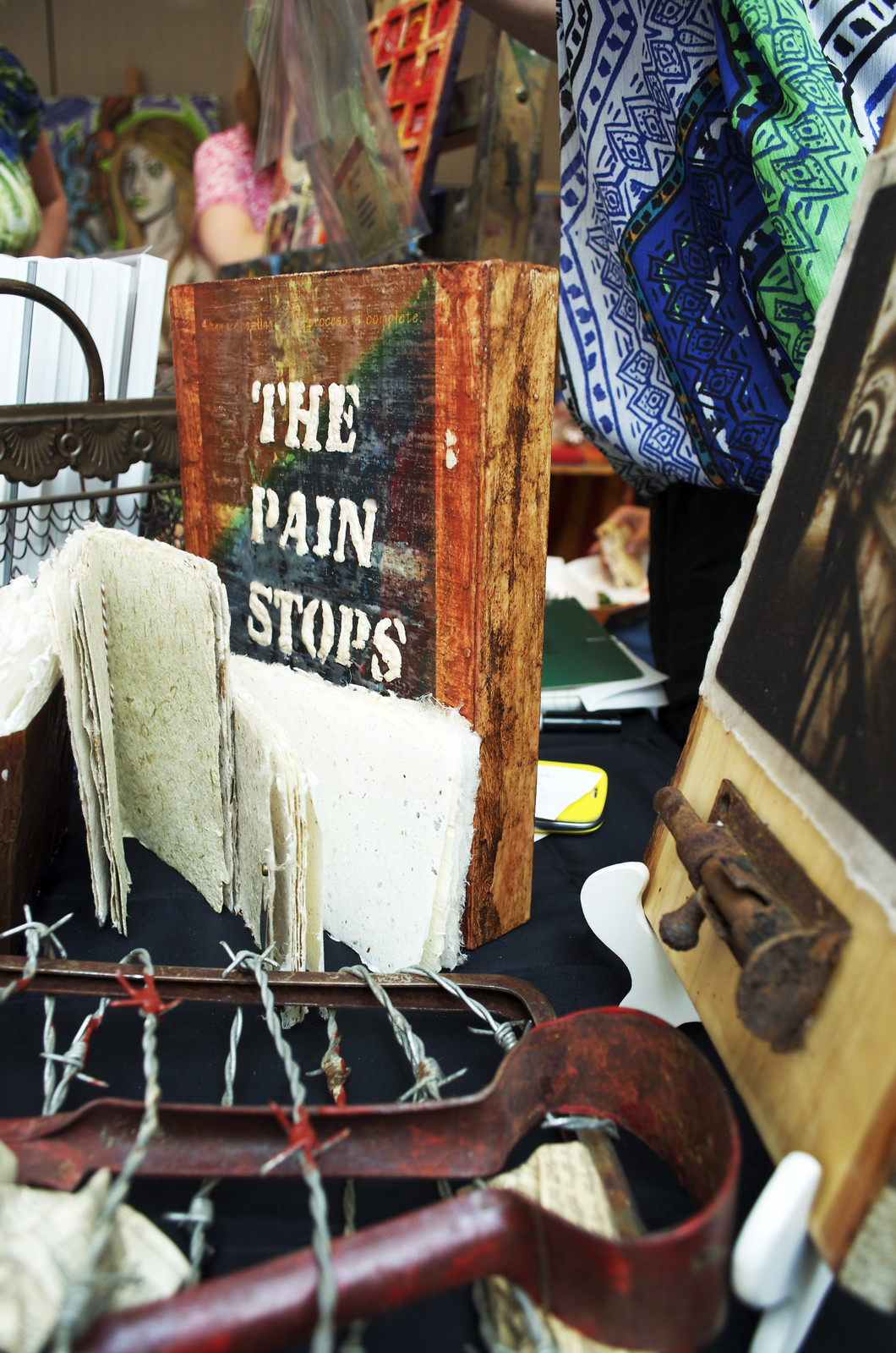This vertically oriented photograph captures a cluttered scene reminiscent of an antique store or flea market. The centerpiece is a black table laden with assorted items, evoking a sense of curated chaos. On the lower left, barbed wire entwines a rusted red clamp, adorned with what appears to be red paint mimicking blood. Above this unsettling object, a book with blank pages or potentially a piece of wood is propped up, bearing the white-lettered phrase, "The Pain Stops." Behind it, a wooden plaque with a bolt lock adds to the eclectic assortment. A colorful scarf in hues of blue, green, and white drapes towards the top of the image, providing a vibrant contrast to the otherwise muted and rustic tones. In the background, various objects, including a painting, further contribute to the tableau of miscellaneous treasures and curiosities. The scene is detailed and rich, reflecting the layered history and stories of the collected items.